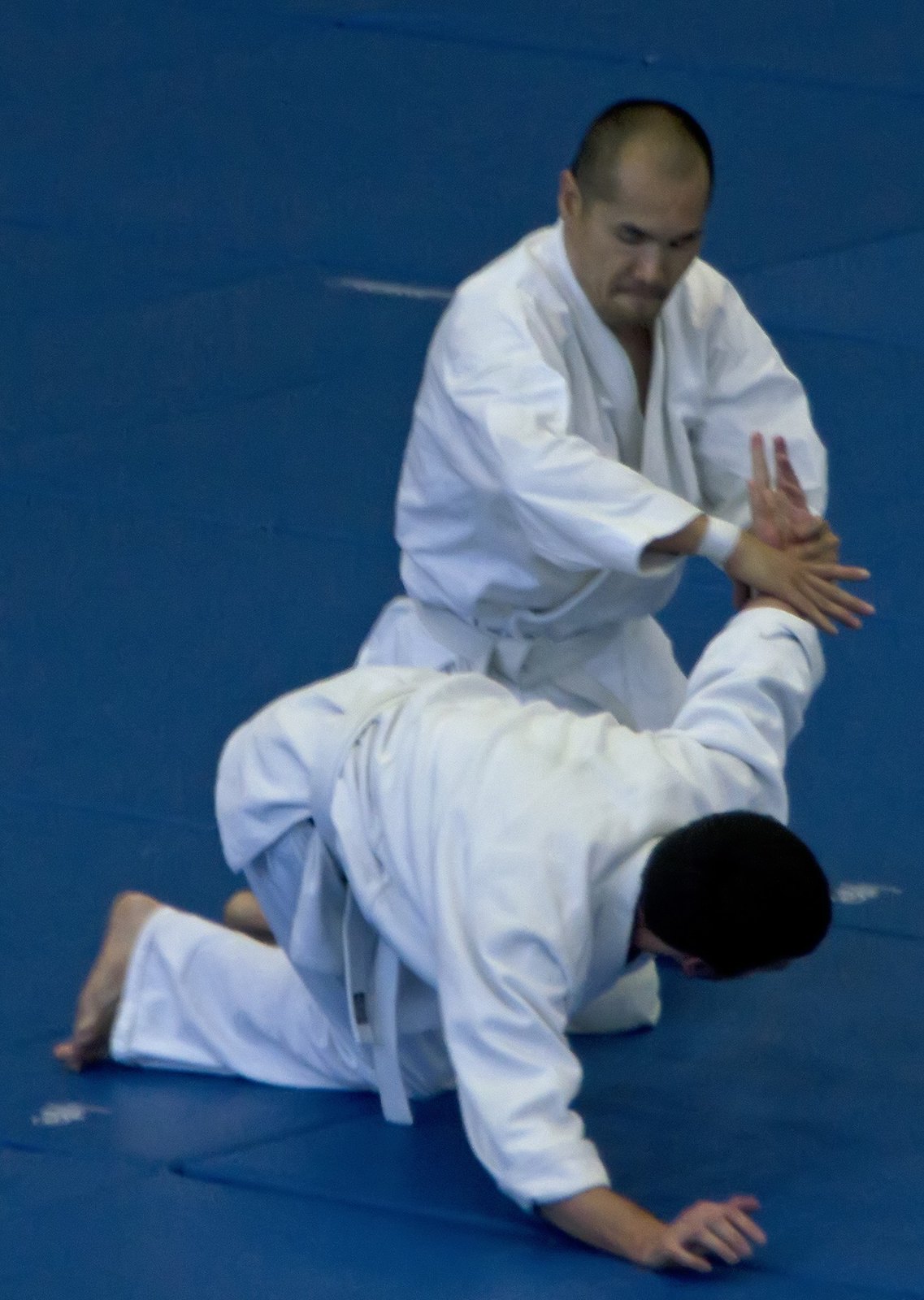The image depicts a martial arts duel between two men on blue gym mats. Both are wearing traditional white martial arts robes. The man closer to the camera is on his hands and knees, his face obscured, with dark hair and barefoot. His left wrist is being forcibly bent backward by the other man, who is a somewhat balding, middle-aged male with short, dark hair and facial hair. This man is standing and gritting his teeth, his attention focused downward as he maintains a firm grip on his opponent's wrist. He is distinguishable by a white wristband on his left wrist. The two are engaged in what appears to be a master-apprentice scenario, with the older man evidently in control. The blue mats below them are segmented, and white lines or markings are visible in various places on the mat.